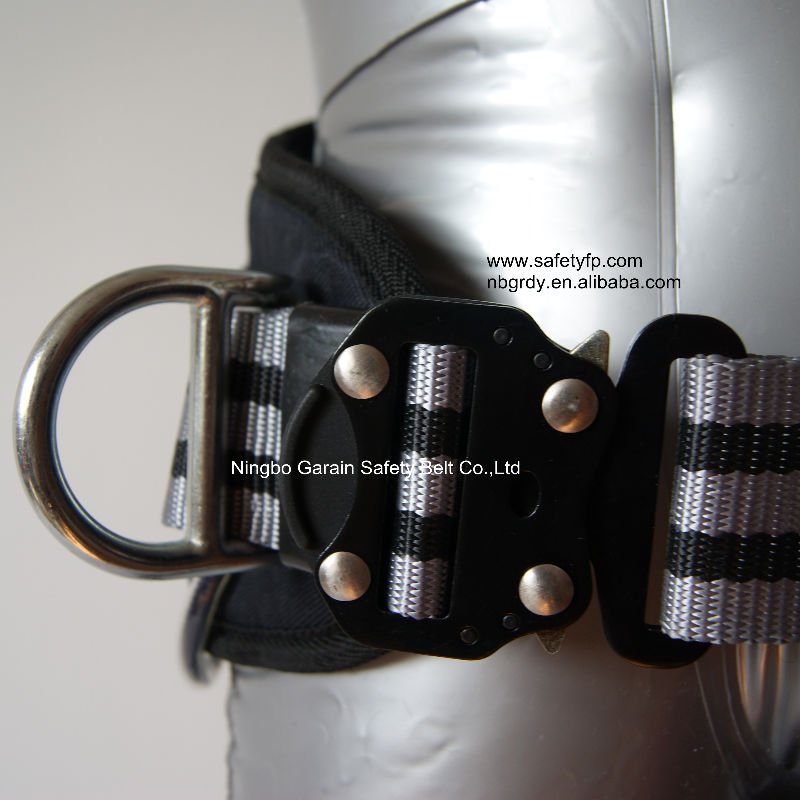The close-up image prominently displays a safety belt from Ningbo Garain Safety Belt Co., Ltd. The belt is silver and black with a metal clasp on the left side. The steel-colored clasp features black hardware secured by four silver bolts, and includes a small round clip for attachments. The belt is wrapped around a soft, silver material that appears to be an inflatable object. Text on the image includes "Ningbo Garain Safety Belt Co., Ltd" in white, approximately size 10 font, with the URLs "www.safetyfp.com" and "nbgrdy.en.alibaba.com" in black, positioned in the northeast quadrant above the belt.